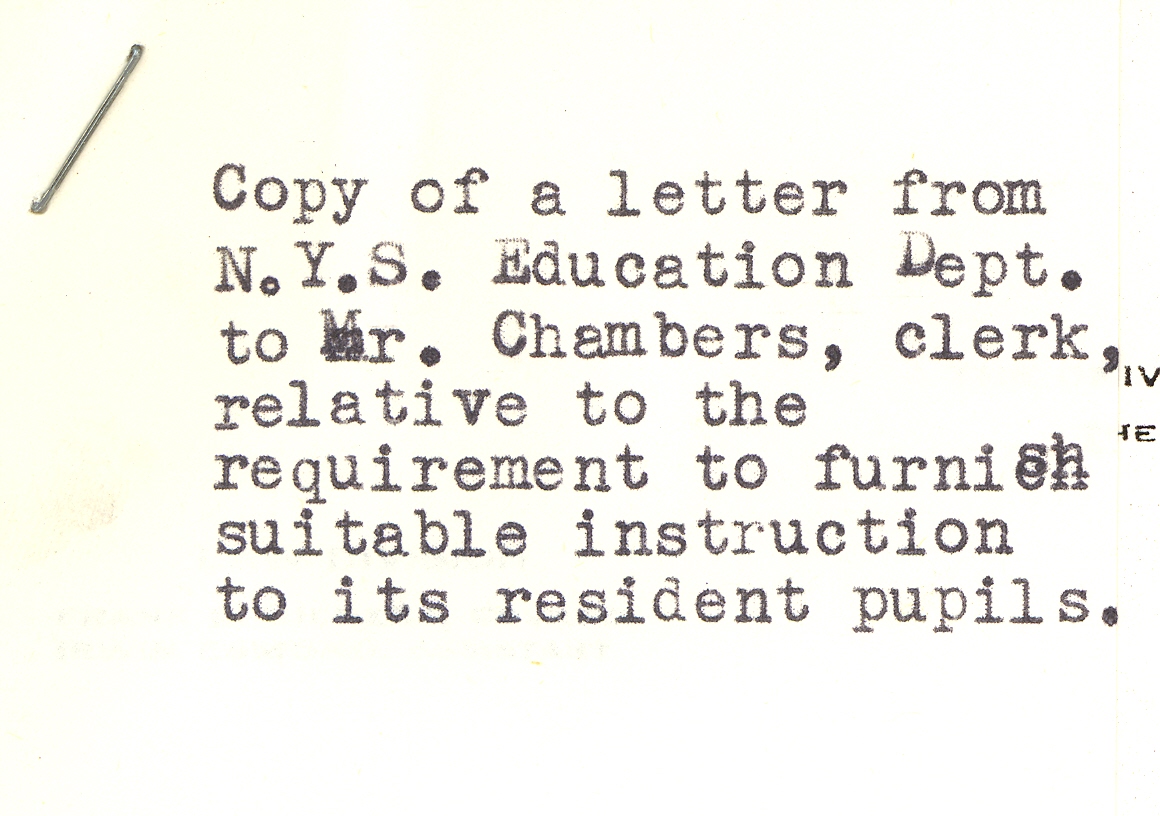The image displays a black and white, horizontally rectangular document that appears to be a typewritten copy of a letter from the NYS Education Department. The background is a very pale yellow, while the typed text is a faded black. The document reads, "Copy of a letter from NYS Education Department to Mr. Chambers, Clerk, relative to the requirement to furnish suitable instruction to its resident pupils." Notable typographical errors include an elevated "D" in "Department" and corrections where "Mr." originally had a lowercase "m" that was overtyped with an uppercase "M." Additionally, "furnish" has an overwritten correction where "CH" was mistakenly typed and "SH" was typed over it. There are also elements in different fonts, such as an "IV" and "IE," which seem to have been added separately. In the left-hand corner, there is a prominent black mark that diagonally spans as though it could represent a misaligned staple, and the text is accompanied by various small typographical inconsistencies.